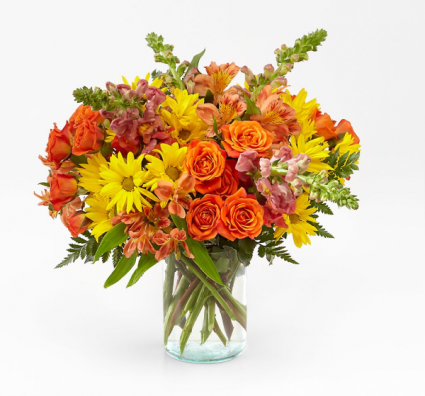This photograph captures a vibrant and abundant bouquet of fresh-cut flowers set against a bright, all-white background. The flowers are arranged in a clear glass jar that resembles a mason jar without any raised writing, filled with water that reveals the bright green stems interspersed with a hint of brown. The bouquet is lavish and varied, featuring warm orange-yellow roses, yellow daisies, and snapdragons, along with other flowers displaying hues of purple-pink and white. Decorative green elements, like ferns and tall grasses, are scattered throughout the arrangement, adding layers of texture and depth. The color palette of the bouquet predominantly features warm yellows, oranges, and peaches, creating a visually stunning and rich composition.